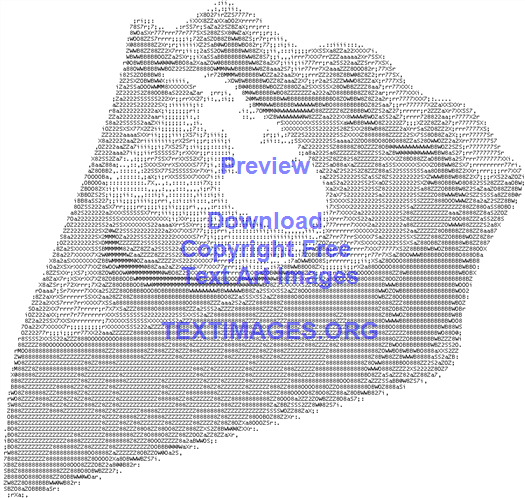The image features a monochrome, text-based depiction of a slice of pie with a dollop of cream on top. The pie, which has a scalloped crust meticulously cut, appears to be crafted using a variety of different numbers and letters arranged without a discernible pattern. Predominantly composed of white text, the image forms a cohesive picture when viewed from a distance. The artwork is overlaid with blue and purple text: at the top, it reads "Preview, Download Copyright Free Text Art Images," and at the bottom, "textimages.org."